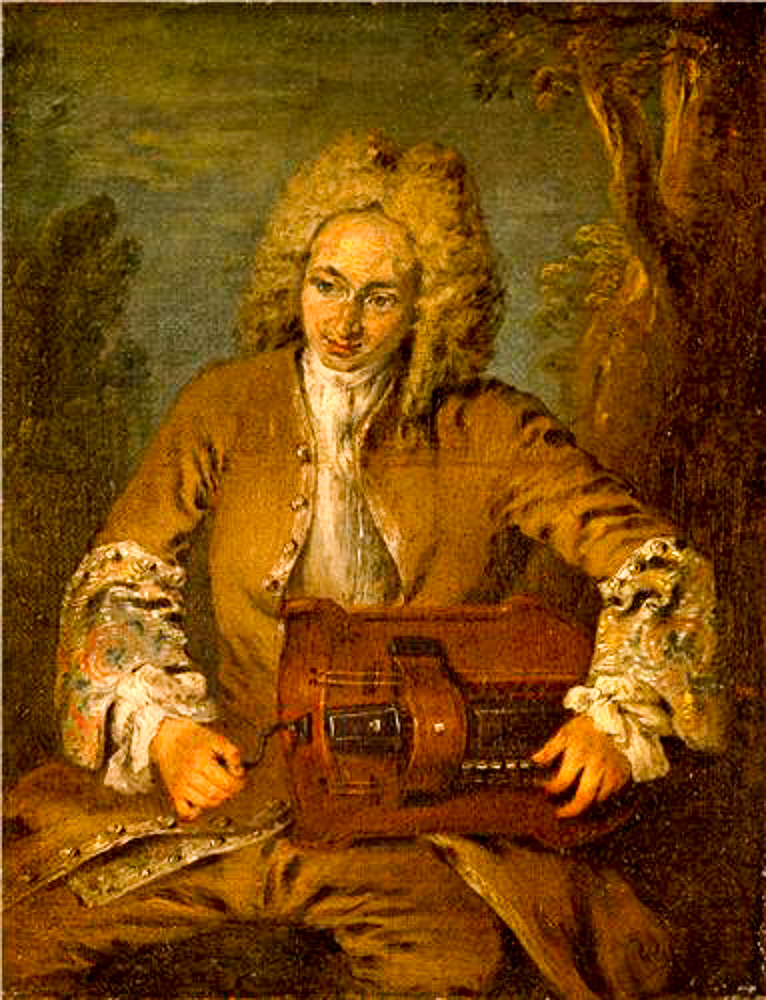The image is an oil painting depicting a man from the 1600s or 1700s, likely an English aristocrat, seated outdoors amidst a natural landscape with visible tree trunks in the background. He wears a noble tan outfit reminiscent of the French Revolution era, complete with a light-colored jacket, embroidered sleeves, and frilled shirt cuffs, paired with matching pants. His long, curly white hair is styled in a powdered wig. The man is playing a wooden musical instrument on his lap that resembles a guitar head but features a turning crank, suggesting it could be a hurdy-gurdy. The overall color theme of the painting is predominantly brown.